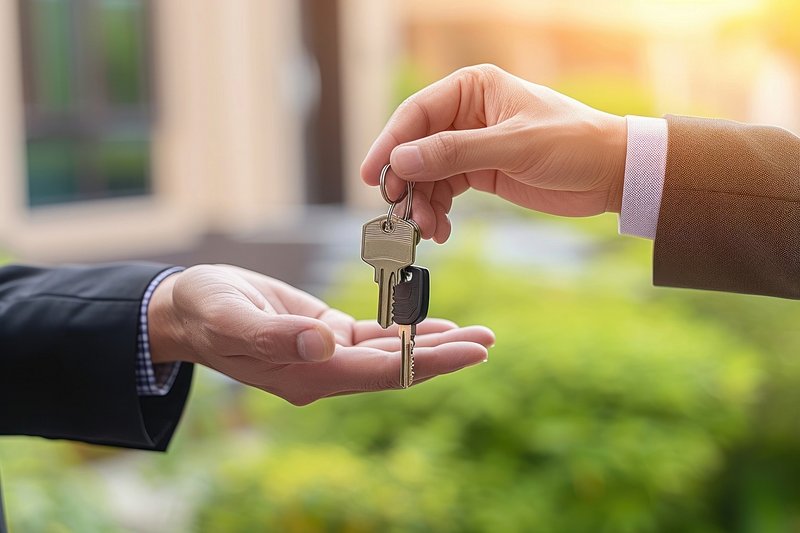This is a close-up, artistically drawn image depicting two male hands engaged in the act of transferring keys. In the center of the composition, one hand, emerging from a dark blue jacket and a blue-and-white checkered shirt, holds a set of two keys—one silver and one black with a silver edge. It is poised above another hand, which is clothed in a brown blazer with a white undershirt, cupped and anticipating the keys. The background is a blur, giving hints of green shrubbery and the exterior of a building, ensuring that the focus remains on the hands and the symbolic exchange.